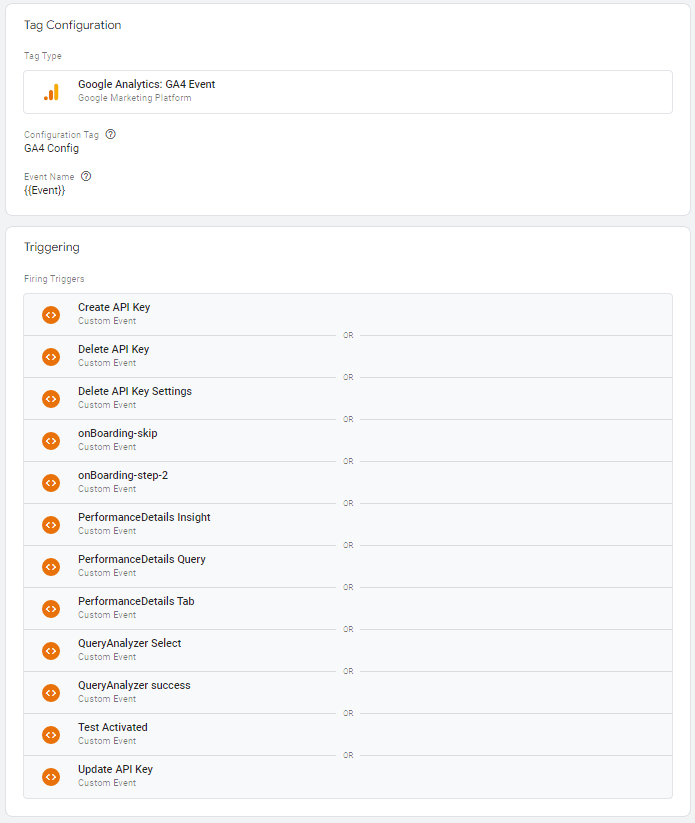This image features a web page centered around Google Analytics configuration and event settings.

In the top left corner, there is a section labeled "Tag Configuration." Directly below this, a sub-section titled "Tag Type" lists three specific options: Google Analytics, GA4 Event, and Google Marketing Platform. 

Within the "Tag Configuration" section, there is a specified type, "GA4 Config," and an "Event Name" field that simply contains the text "event" enclosed in brackets.

Beneath this configuration area, another table labeled "Triggering" appears in the top left corner, followed by "Firing Triggers." This table presents a list of twelve options:
1. Create API Key
2. Delete API Key
3. Delete API Key Settings
4. Onboarding Skip
5. Onboarding Step Two
6. Performance Details Insight
7. Performance Details Query
8. Performance Details Tab
9. Query Analyzer Select
10. Query Analyzer Success
11. Test Activated
12. Update API Key

Each of these options is indicated by an orange circle with white lines, suggesting selectable triggers for configuring specific behaviors.

Overall, the page provides a clear interface for setting up and managing various aspects of Google Analytics, confirming the use of the Google Analytics platform, particularly its GA4 configuration capabilities.